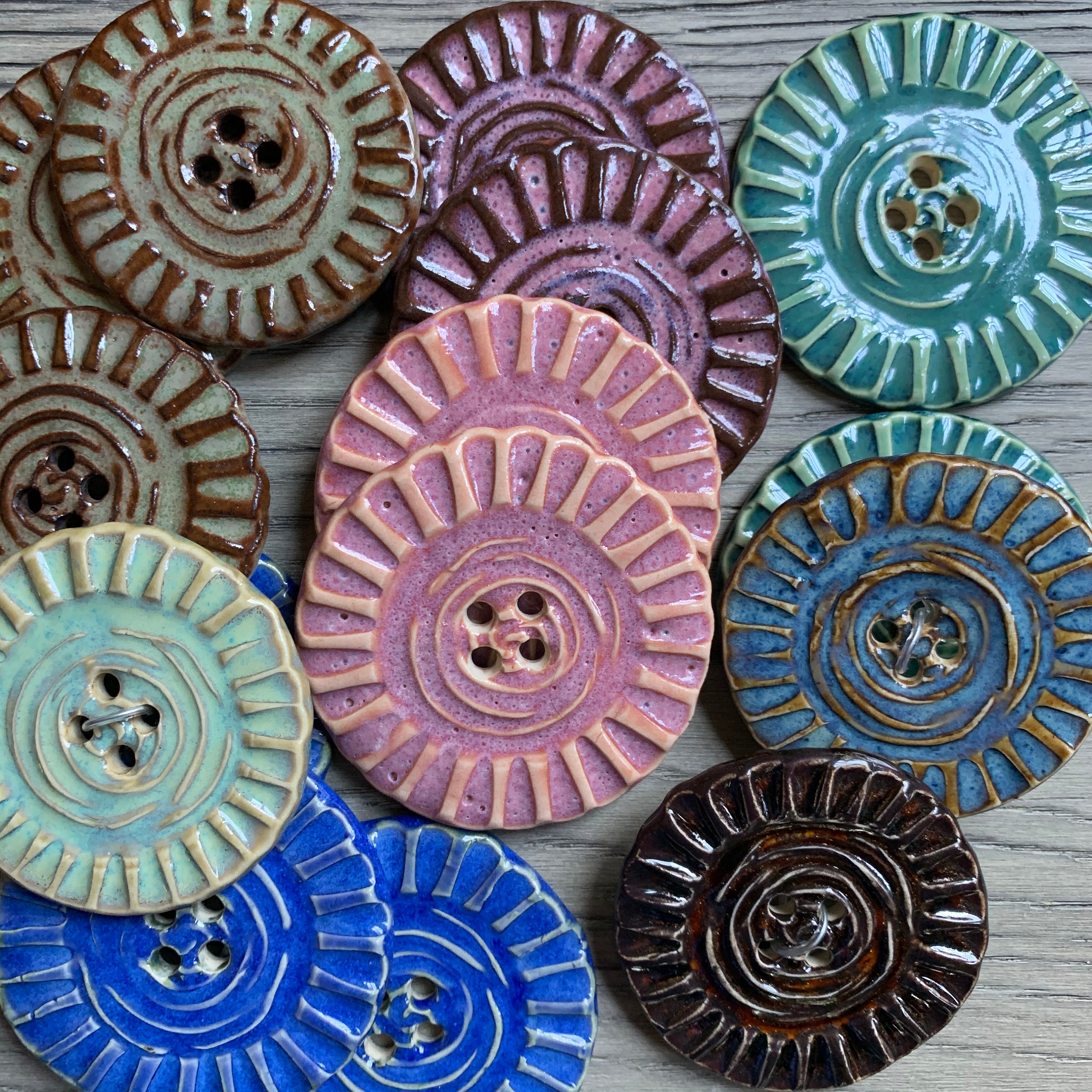This image is a detailed color photograph of a small pile of ornate, handmade two-inch ceramic buttons, arranged randomly on a grayish white woodgrain background. Each button, designed with four holes in the center for sewing onto garments, features a unique color and intricate decorative patterns. The designs include a range of colors from earthy browns with grayish undertones, to mauve pink and gold with seafoam blue backgrounds, to deep royal blue and hunter green. A light green button with brown hash marks sits in the top left, while two lavender buttons with dark purple designs are positioned in the top center. An aqua button with light green decoration is in the top right. Additionally, there are a single mint green button with cream decorations, pink buttons with light cream markings stacked vertically in the center, a medium blue button with gold highlights, a black button with white details, and two bright blue buttons with similar white decorations. The buttons are characterized by their smooth, textured ceramic surfaces, detailed with outward grooves forming borders and circular inner lines.